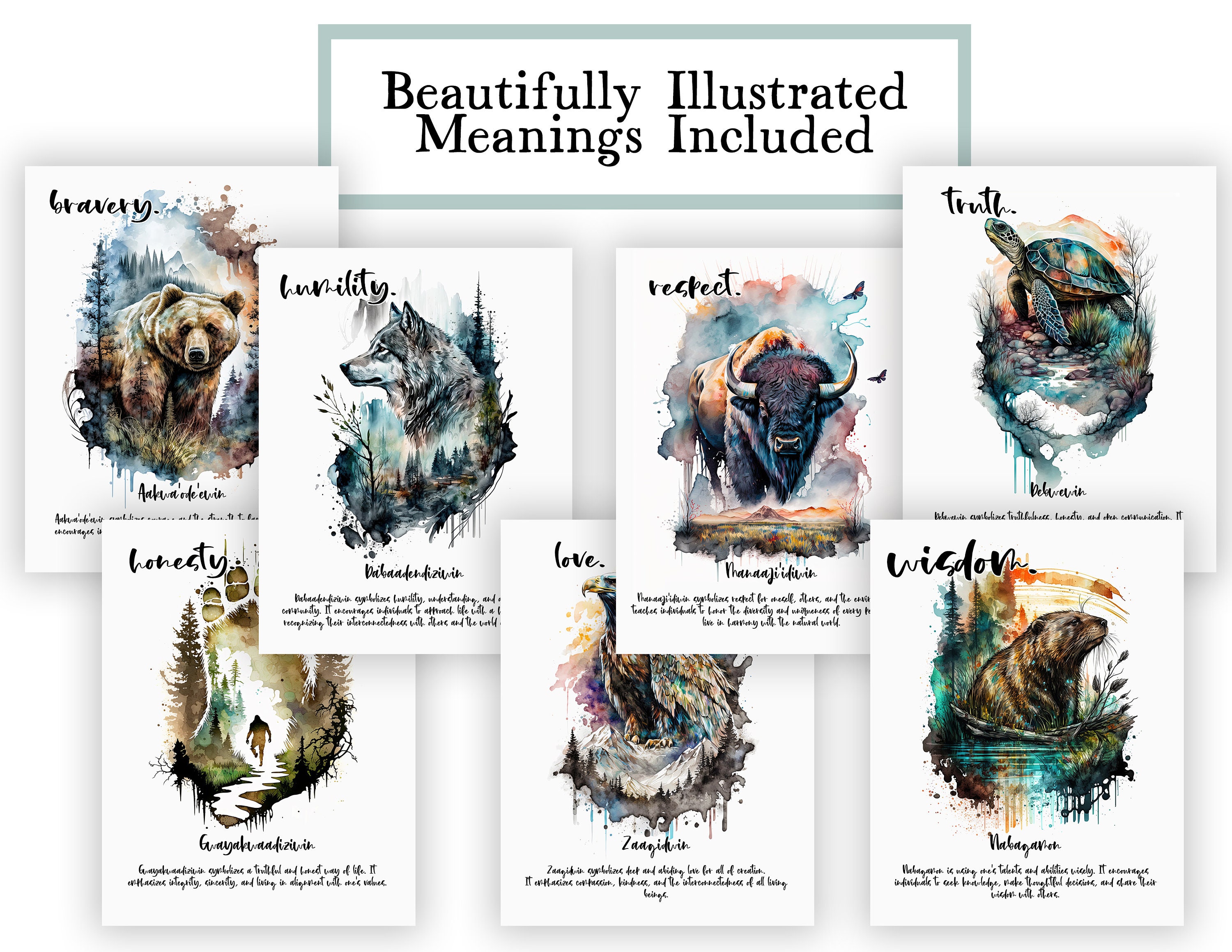The image depicts seven beautifully illustrated watercolor paintings of wildlife, each accompanied by a word and a small, somewhat difficult-to-read text beneath them. At the top center, a blue-bordered box states "beautifully illustrated meanings included." 

1. **Bravery:** The upper left painting features a grizzly bear in brown coloring, set against a backdrop with mountains, fir trees, and grasses.
2. **Humility:** Next is a gray wolf looking stoically to the left, with trees painted below it.
3. **Respect:** The third painting shows a light tan buffalo with a reddish-brown face and forward-facing horns.
4. **Truth:** This illustration features a light green turtle with a dark green shell, its neck extended upward.
5. **Honesty:** Portrayed in the bottom left, this image seems to depict a Sasquatch or Bigfoot-like creature walking through a forest path.
6. **Love:** An eagle, likely a golden or bald eagle, is shown gazing skyward, though it is partially obscured.
7. **Wisdom:** The final painting features a small rodent-like creature, possibly a beaver, gopher, or otter, looking ahead.

Each painting is framed with elements of the animal's habitat, rendered in a soft, flowing watercolor style, creating a cohesive and themed set of art pieces.